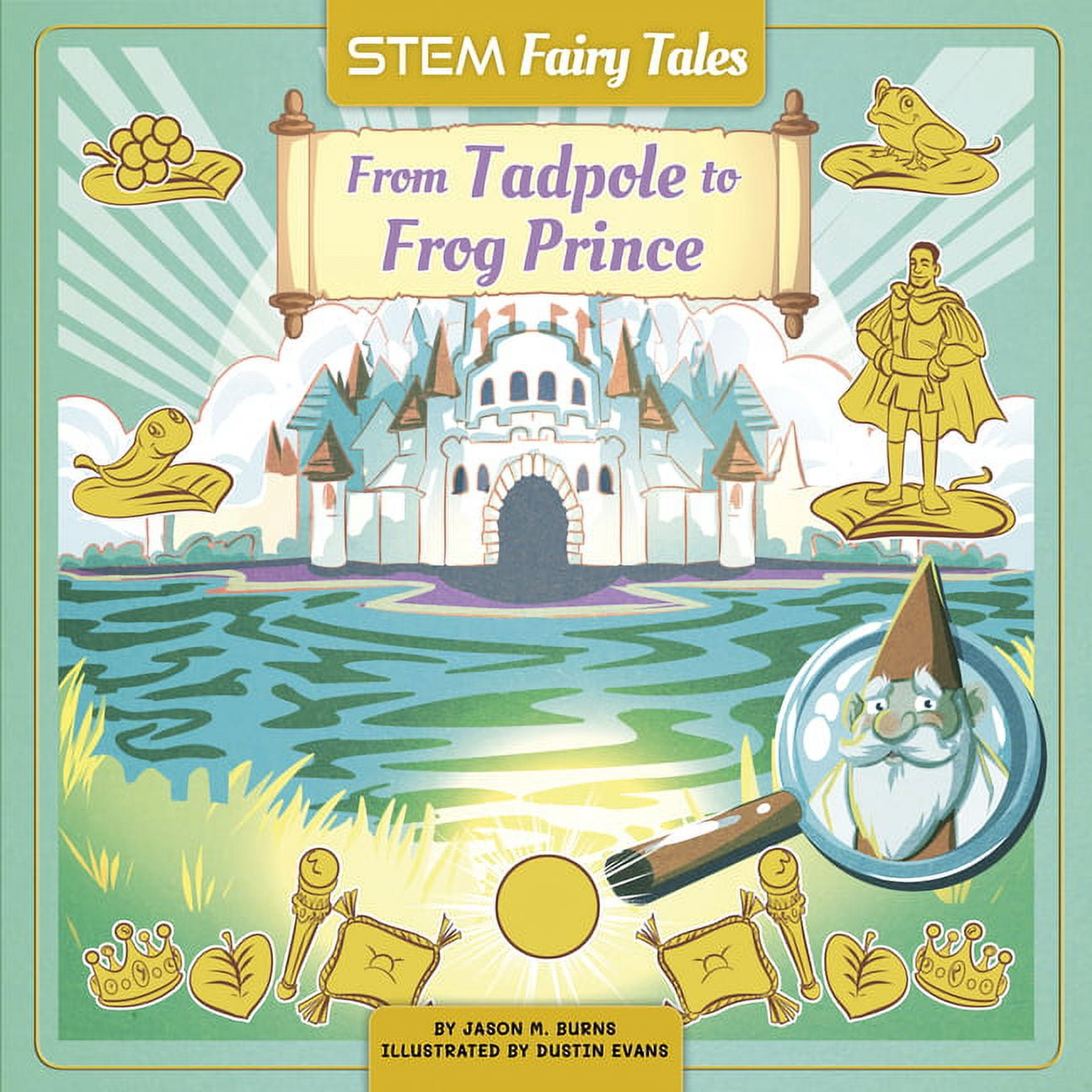The cover of this children's book, aimed at introducing STEM education to younger kids, is an eye-catching blend of fantasy and learning. Set against a mint to grass green background, the top portion of the cover features a golden banner with "STEM Fairy Tales" written in crisp white text. Below that, a tan scroll with purple text reveals the title, "From Tadpole to Frog Prince." Authored by Jason M. Burns and illustrated by Dustin Evans, the cover showcases a majestic white castle prominently centered. Surrounding the castle are various elements tied to the story's theme and fairy-tale royalty: a gleaming crown, scepters, plush pillows, a lily pad, and numerous golden figures including a frog, a snake, a prince, and what seems to be a fish. Also depicted are stages of a frog's lifecycle—eggs on a leaf, a tadpole, and a frog—highlighting the book's educational aspect. At the bottom right, a magnifying glass encases a whimsical gnome, adding to the enchanting allure of the cover. Water elements and assorted imagery further encapsulate the magical yet informative nature of this captivating book cover.